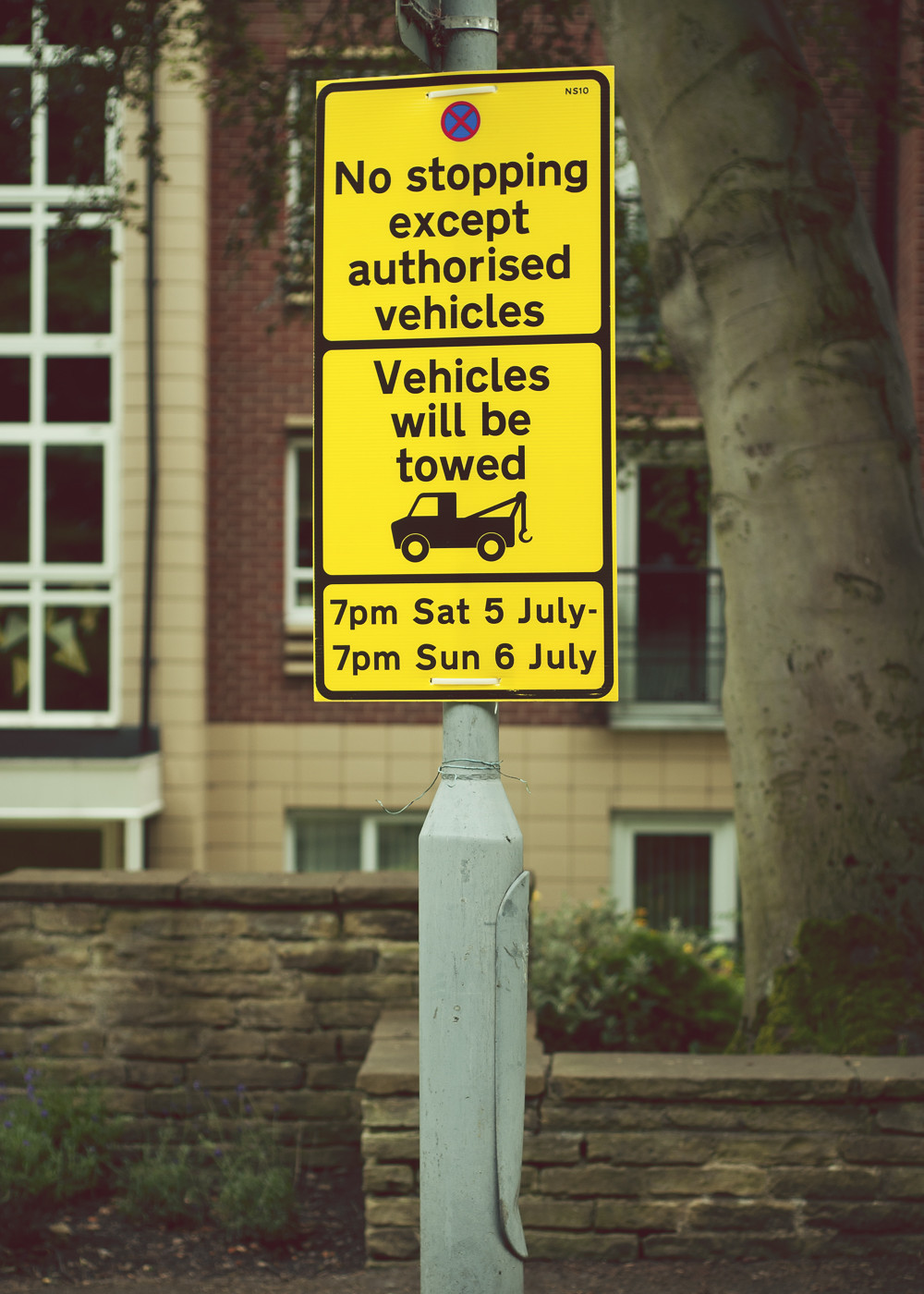The photograph, taken outdoors on an overcast day, captures a detailed street scene with a prominent yellow sign affixed to a white metal pole at its center. This sign, divided into three sections outlined in black, features a red circle with a red X on a blue background at the top, symbolizing restricted parking. Below it, black text reads, "No stopping except authorized vehicles." The middle section warns, "Vehicles will be towed," accompanied by an illustration of a tow truck. The bottom section gives specific towing times: "7 p.m. Saturday, 5th of July through 7 p.m. Sunday, 6th of July." The backdrop includes multi-story buildings—one tan with white windows, the other red brick, also with white windows—alongside a large tree growing from a slabbed planter that doubles as seating. The foreground features a retaining wall made of tan bricks and a sidewalk, encapsulating the everyday urban environment.